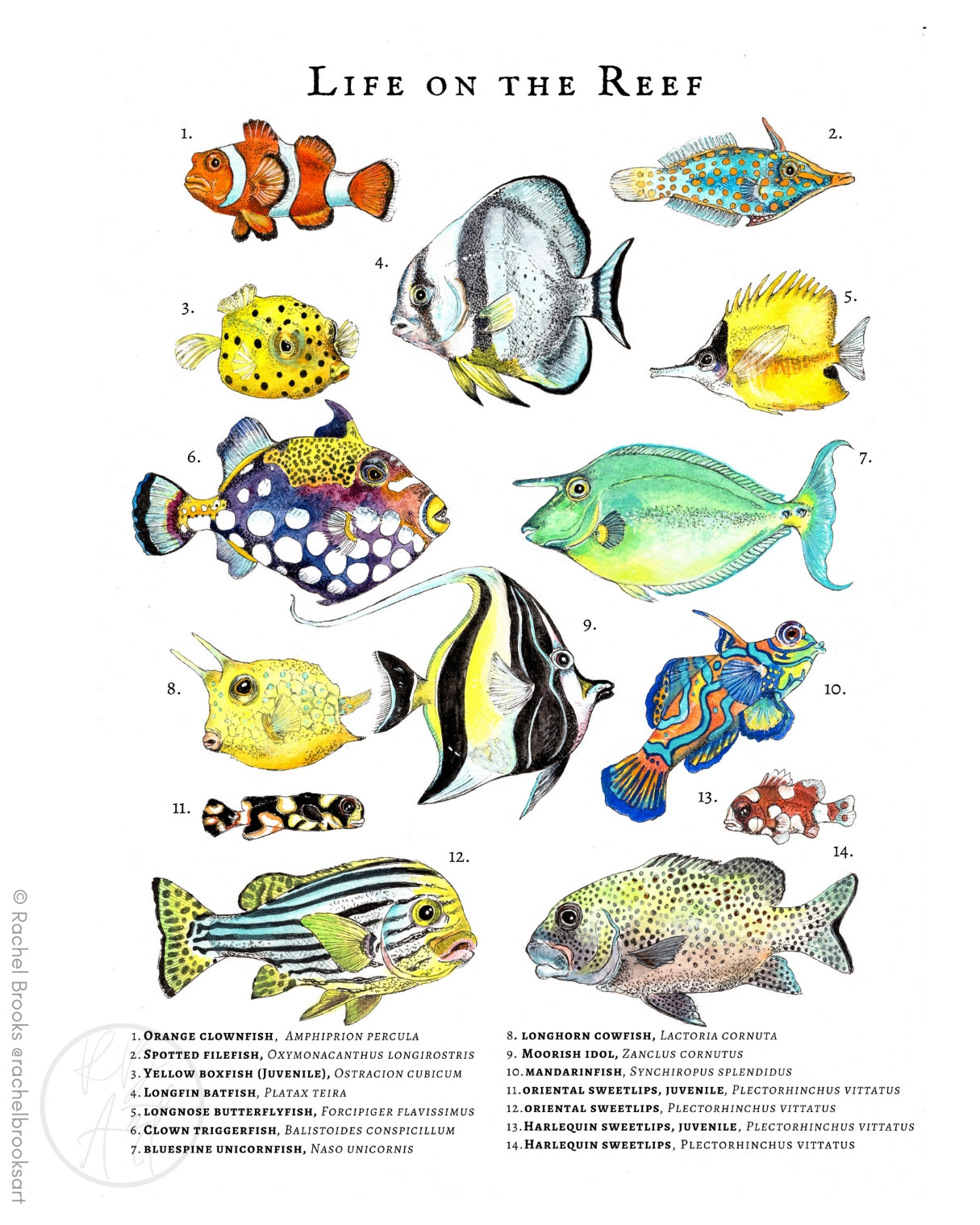The image is a detailed, color diagram titled "Life on the Reef," showcasing 14 different fish species living near the reef. Set against a white background, each fish is beautifully illustrated in vibrant colors and varying sizes and shapes. The fish are numbered one through fourteen, with their names and scientific names printed in black text at the bottom. Among the fish depicted are:

1. **Orange Clownfish** - Orange with white stripes.
2. **Spotted Filefish** - Blue and orange polka dots with a long nose.
3. **Yellow Boxfish Juvenile** - Yellow with black polka dots.
4. **Longfin Batfish** - Black and white striped, clove or spade-shaped body.
5. **Longnose Butterflyfish**
6. **Clown Triggerfish**
7. **Blue Spine Unicornfish**
8. **Longhorned Cowfish**
9. **Moorish Idol**
10. **Mandarin Fish**
11. **Oriental Sweetlips Juvenile**
12. **Oriental Sweetlips**
13. **Harlequin Sweetlips Juvenile**
14. **Harlequin Sweetlips**

The artwork is credited to Rachel Brooks, with her name positioned at the bottom left corner from top to bottom. Each fish is meticulously depicted, creating an educational and visually appealing representation of reef life.